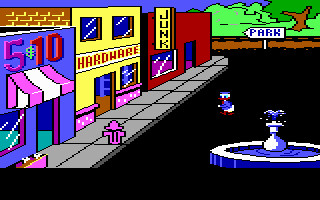In this vibrant arcade game scene, players find themselves in a colorful street bustling with character and charm. The street features a variety of shops, each with distinct architectural styles and bright hues. To the left, there’s a brilliant blue building adorned with a pink awning, its sign prominently displaying a price of $5 and the number 10. Nearby, a yellow storefront stands out with the word "Hardware" emblazoned in bold red letters. On the right, a striking red building, marked "Junk" in eye-catching yellow, adds to the eclectic mix. Amid these shops, a sign with "Park" in bold lettering points to the left, leading to an area filled with lush trees and other natural elements.

The street itself is a stark contrast, paved entirely in black, providing a dramatic stage for a whimsical duck character dressed in a sophisticated suit. This dapper duck appears to be walking toward the sidewalk, intent on entering one of the inviting stores. Completing the scene, a serene water fountain is situated at the very bottom right of the image, adding to the ambiance and charm of the arcade game’s setting.